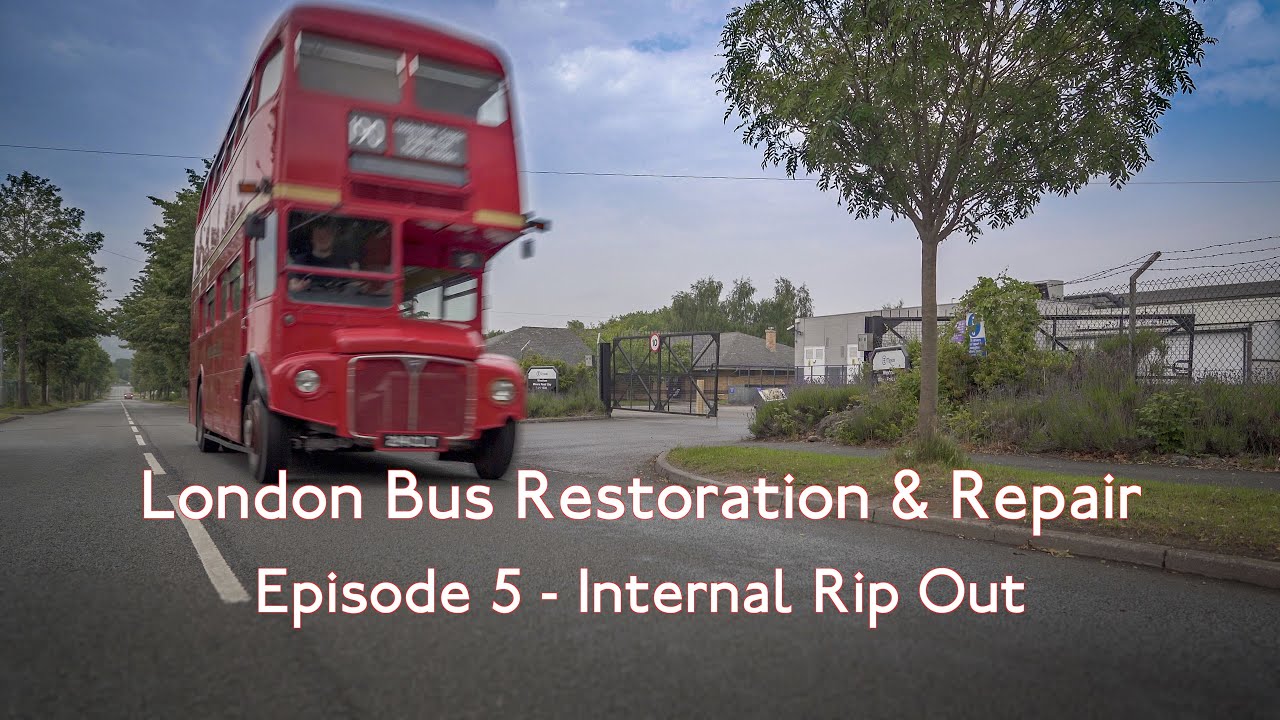The image appears to be a thumbnail or a screenshot of a video titled "London Bus Restoration and Repair, Episode 5, Internal Ripout." The central subject of the picture is a slightly blurry, double-decker red bus in motion, situated in the right lane of a grey road marked with white dotted lines. The bus, displaying a British license plate, is advancing towards the viewer. 

The photo captures a commercial zone in the background, featuring a white warehouse with a large black sliding gate. The surrounding yard is enclosed with fencing topped with barbed wire. Trees bracket both sides of the road and a sidewalk runs parallel on the right side of the image. The sky is a clear blue dotted with white clouds. Overlaying the image, white text at the bottom reads, "London Bus Restoration and Repair, Episode 5 - Internal Ripout." The scene suggests this is part of a series, likely a YouTube video, focused on the restoration of classic London buses.